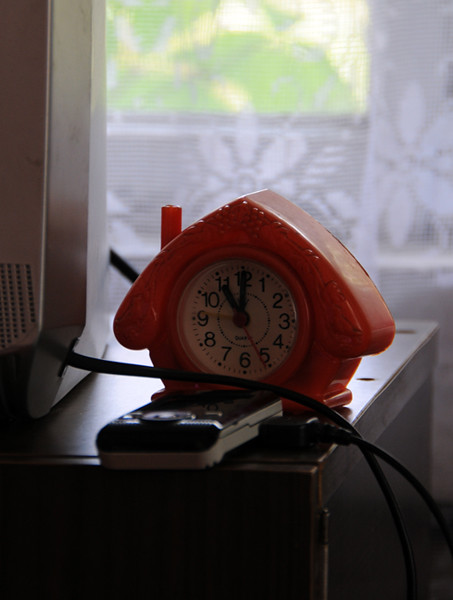The image portrays a cozy bedside table positioned in front of a window adorned with sheer, floral-patterned net curtains. Through the curtains, the green hues of a garden are faintly visible. The bedside table is a dark brown, rectangular piece of furniture. On it stands an eye-catching alarm clock, designed whimsically in the shape of a small red house. The clock, made of a rubbery plastic, features a white clock face with large, bold black numbers ranging from 1 to 12, and has child-like elements, possibly to help in learning to read the time. This clock has a distinctive triangular roof and a small chimney, and its hands include two black ones for hours and minutes, as well as a thin red second hand pointing past five. In front of the clock is a phone plugged in and charging, its cable coiled neatly. To the right of the clock, a small portion of a silver rectangular object, presumably a TV, peeks into the frame.